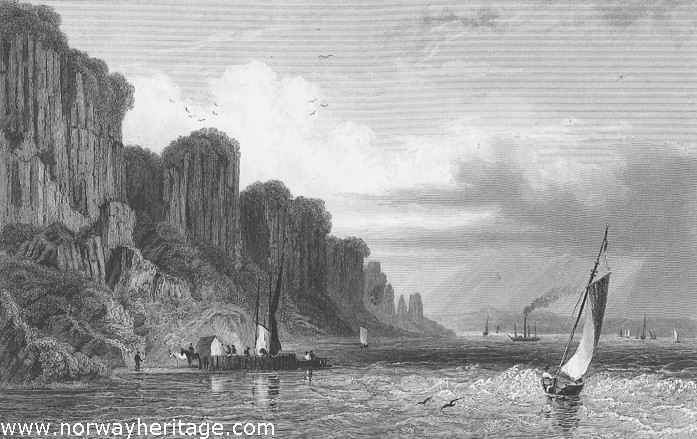This detailed monochrome drawing from NorwayHeritage.com portrays a historic maritime scene set against a rugged shoreline, likely in Norway. Prominent on the left are steep, rocky cliffs that descend into a lively body of water dotted with various vessels. In the foreground, a sailboat approaches a dock that appears to be supported by wooden logs. To the right of the sailboat stands a smaller boat and further out are additional vessels, including a distinctive steamship emitting smoke from its chimney. Near the shoreline, we observe a house and a man with a horse, suggesting a daily life scene. The sky has a few birds and clouds, with sunlight filtering through the top right corner, adding a serene touch to the overall composition. This drawing, seemingly a historical reproduction, captures a vibrant yet tranquil day by the sea.